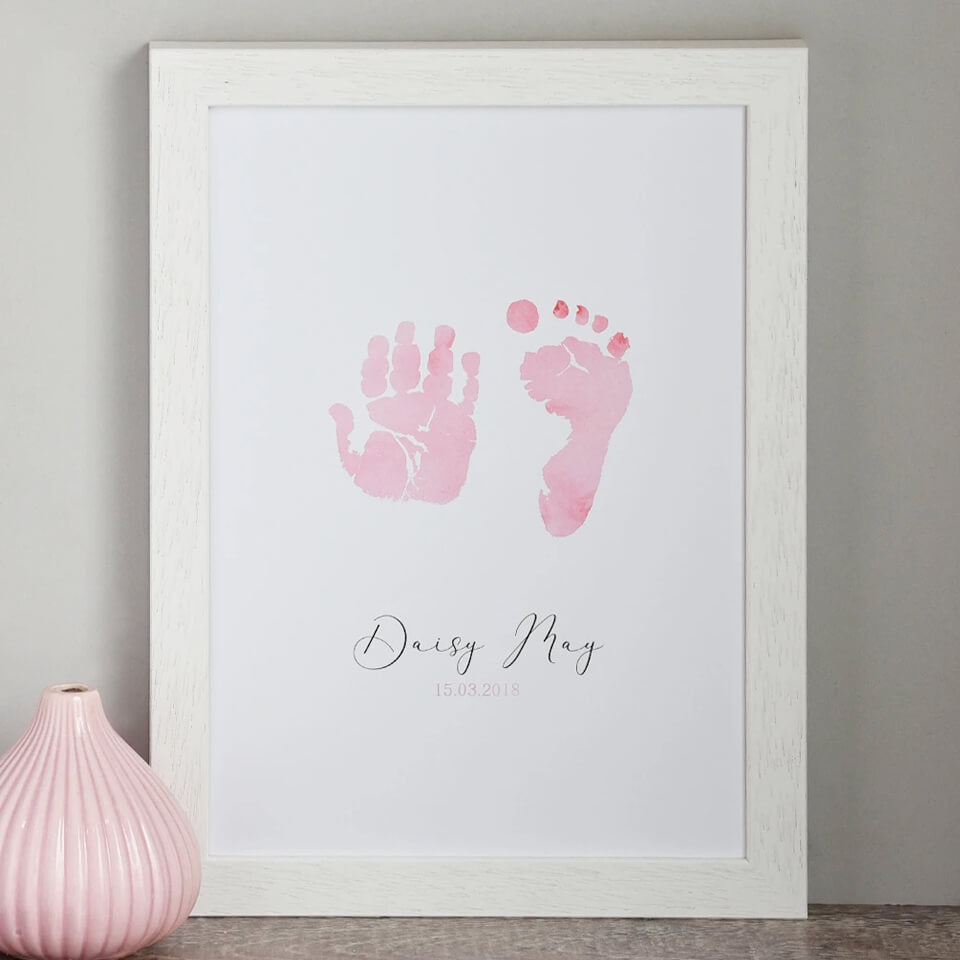In this portrait-oriented photograph, the primary focus is a framed picture leaning against a white wall. The frame itself is made of white wood and rests on a slightly darker brown wooden table. Within the frame, set against a white background, are a small pink handprint on the left and a small pink footprint on the right, both created with pinkish-purple ink. Below these prints, in elegant cursive black lettering, reads the name "Daisy Mae." Further below, in light pink text, is the date "15.03.2018," which likely represents a birthdate. To the lower left and partially in front of the frame sits a small ceramic vase, light pink in color and shaped somewhat like an onion with a pointed top, seemingly placed there to prevent the frame from slipping.